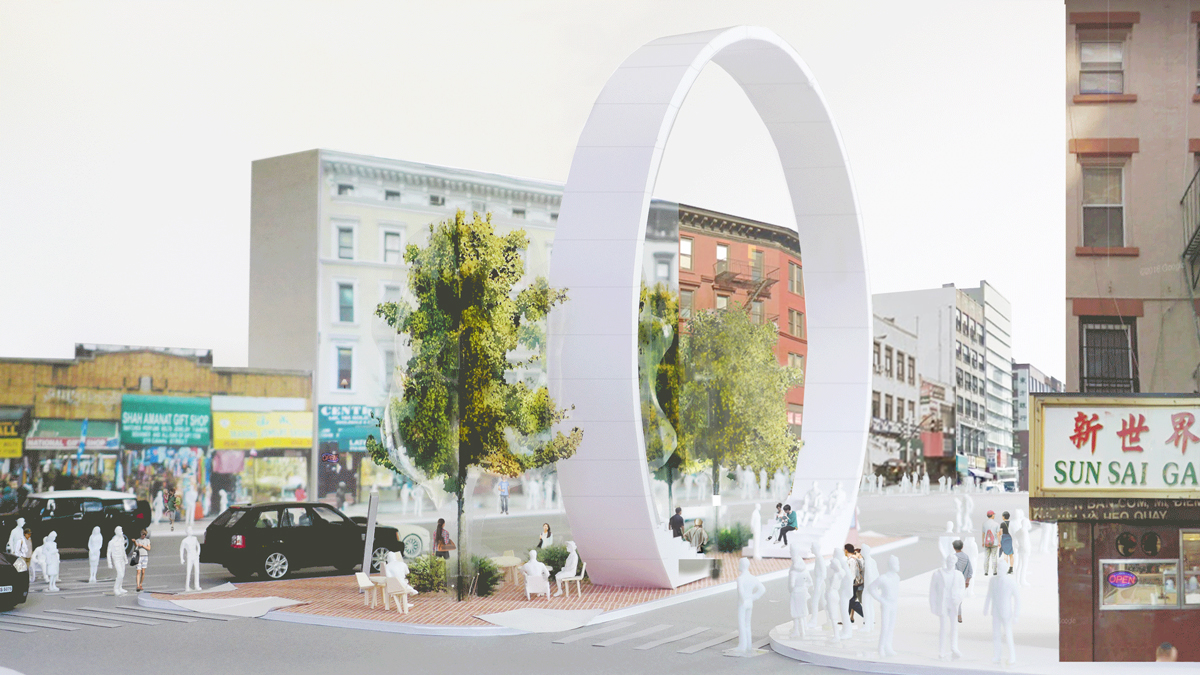The photograph, taken outdoors during the daytime, features a city square in an Asian downtown area under dull natural light, giving the scene a subdued, non-vibrant atmosphere. The square is populated with numerous strikingly white statues of people, positioned as if they are standing at street corners, sitting on benches, or milling about—almost blending into the background due to their stark whiteness. Among these statues, real people can be seen, dressed in dark blue or other colored clothing, mingling with the figures. Central to the square is a large, white arch-like structure that resembles the Gateway Arch in St. Louis and stretches skyward. This arch, described as a big zero or a giant loop, is situated over a median filled with benches and chairs where people can sit and observe the traffic. In the lower right-hand corner of the scene, there's a sign with red Asian characters and green Roman letters that reads "Sun Se Gai," situated above a brown building. The square's layout and the combination of real people and artistic white silhouettes create an almost surreal, artistic impression.